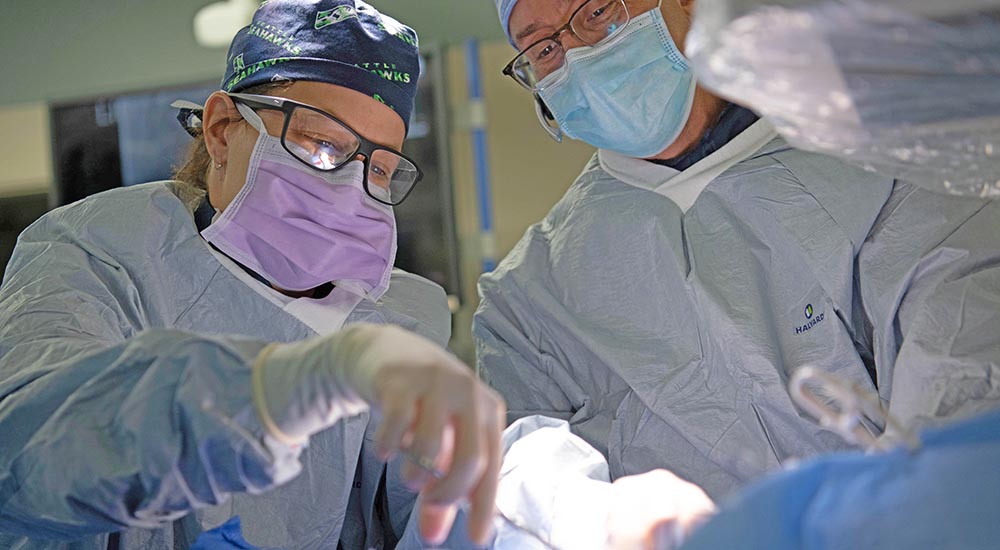In a brightly-lit hospital operating room, two doctors are intently focused on performing surgery. The scene is vivid with the colors of periwinkle, lilac, beige, various shades of gray, charcoal, and white, which are prominently featured in the room and attire. The female doctor, situated on the left, is wearing blue scrubs, a purple mask, black-framed glasses, and a cap adorned with the logo of the Seattle Hawks sports team. She is meticulously handling surgical instruments with gloved hands. On the right, the male doctor is dressed in similar blue scrubs, a blue mask, and glasses that have no bottom frame. Both doctors have their heads covered with surgical caps and appear thoroughly professional in their demeanor. The male doctor, particularly, seems very pleased as he assists in the surgery. Although the patient is not visible in the frame, the setting unmistakably conveys the seriousness and precision typical of an operating room.